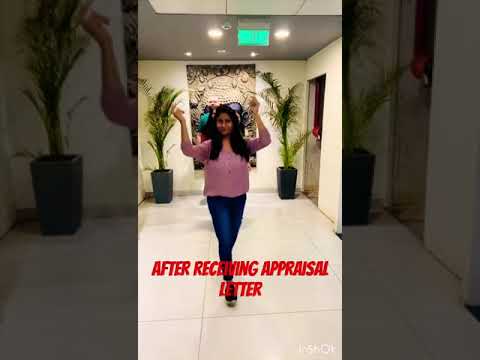The image captures a joyful moment of a young woman with dark hair and a brown skin tone, celebrating after receiving an appraisal letter, as indicated by the red text along the bottom of the image. She is wearing blue jeans, white sneakers, and a long-sleeve pink top as she walks forward with her arms raised at right angles, a broad smile on her face. The scene is set inside a building, possibly a hotel, with a white tiled floor and white walls. In the background, there is an open doorway flanked by two potted plants housing tall green ferns or palm trees, almost reaching the ceiling. A person wearing a green and black shirt stands to her left. Additional details include a beige 3D wall art behind her, recessed lighting, and a green hanging sign from the ceiling.